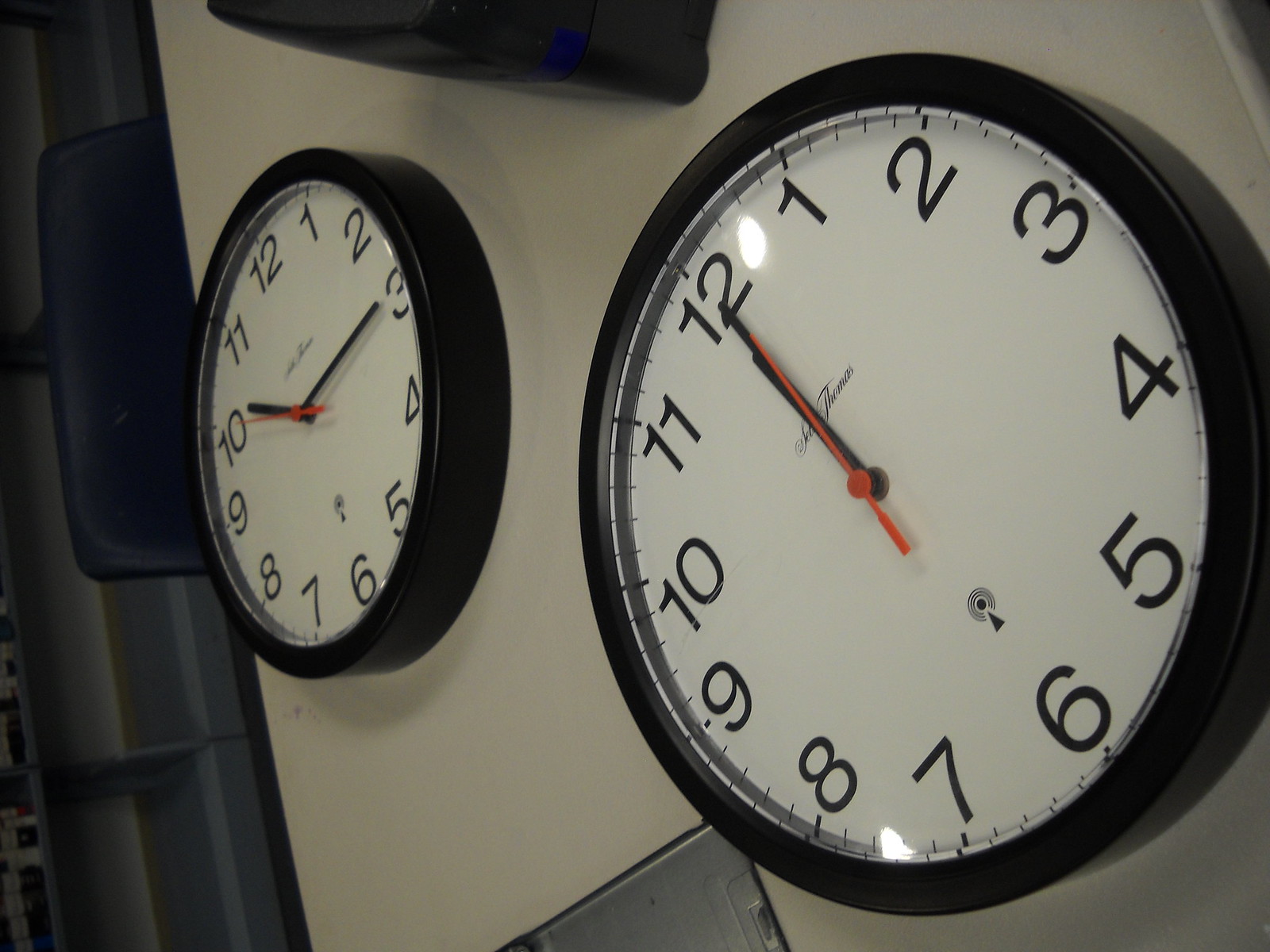This photo showcases two identical round wall clocks with black cases mounted against a stark white wall. Both clocks feature a white face adorned with black numerals, and their brand, something Thomas, is printed just below the '12' on each clock. Notably, both clocks have black hour and minute hands, while their second hands are a contrasting red. The lower clock prominently displays the time as exactly 12 o'clock, while the upper clock, positioned diagonally to the left, indicates the time as 10:15. A subtle reflection of overhead lights can be seen in the glass face of the lower clock, adding an additional layer of detail to the composition.